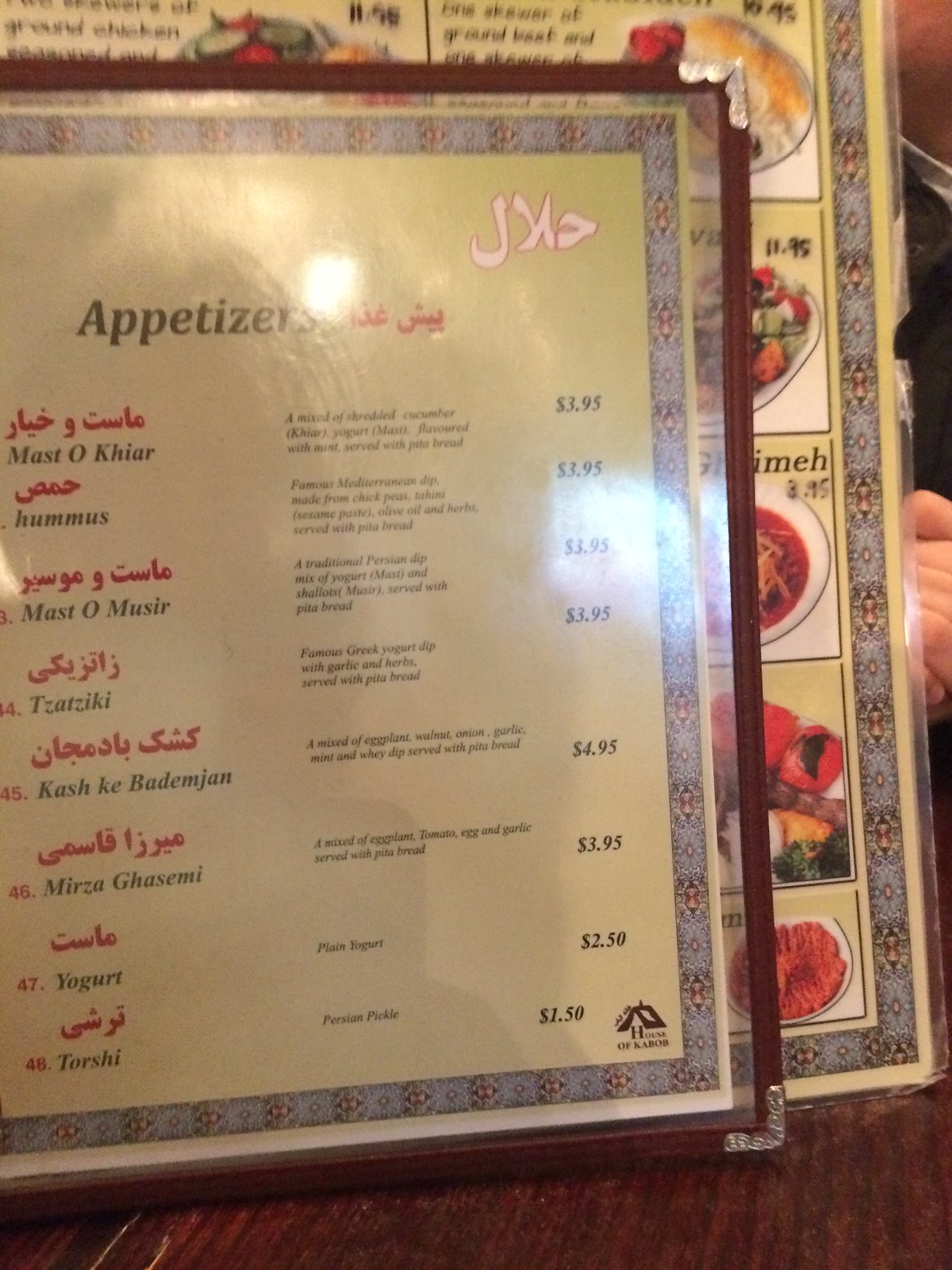This image captures a detailed view of a restaurant's menu, focusing primarily on the appetizers section. The foreground features a page labeled "Appetizers" written in both English and what appears to be a Middle Eastern or Mediterranean language. The listed items include popular dishes such as hummus, tzatziki, myrza, and yogurt. Notably, the prices are quite reasonable, suggesting that the menu might be from a past era. Behind this page, a larger menu page is visible, showing the edges at the top and right side. This second page contains pictorial representations of various entrees, offering a visual guide to the menu items. The appetizers section on the foreground page lists around eight or nine choices, with prices ranging from $1.50 to $4.95.